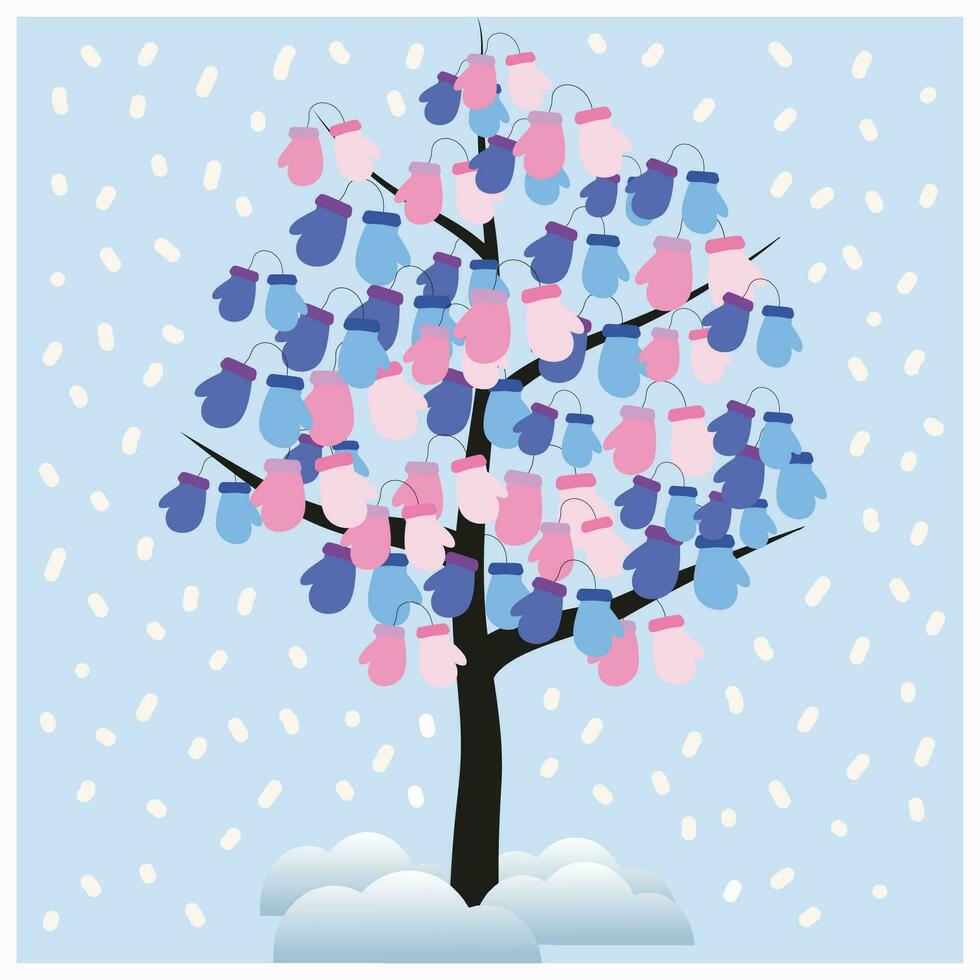This digital vector illustration resembles a whimsical postcard with a snowy, winter theme. The background is a very light blue, suggestive of a cloudy sky, and features scattered white shapes reminiscent of falling snowflakes and sprinkles. Dominating the image is a simplified tree with thin, black branches spreading out from a slender trunk. The base of the tree appears to rise from puffy, greyish-white clouds. 

Instead of leaves, the branches are adorned with dozens of colorful mittens, creating the illusion that the mittens are the tree's foliage. The mittens come in a variety of hues, including dusky blue, light blue, various shades of pink, and purple. Some mittens are mismatched yet connected by strings, with pairs like dusky blue and light blue, or pink and white, repeating throughout the tree. A white border frames the illustration, enhancing its postcard-like appearance. The scene exudes a charming, festive atmosphere, akin to a mitten-decorated Christmas tree amidst a gentle snowfall.